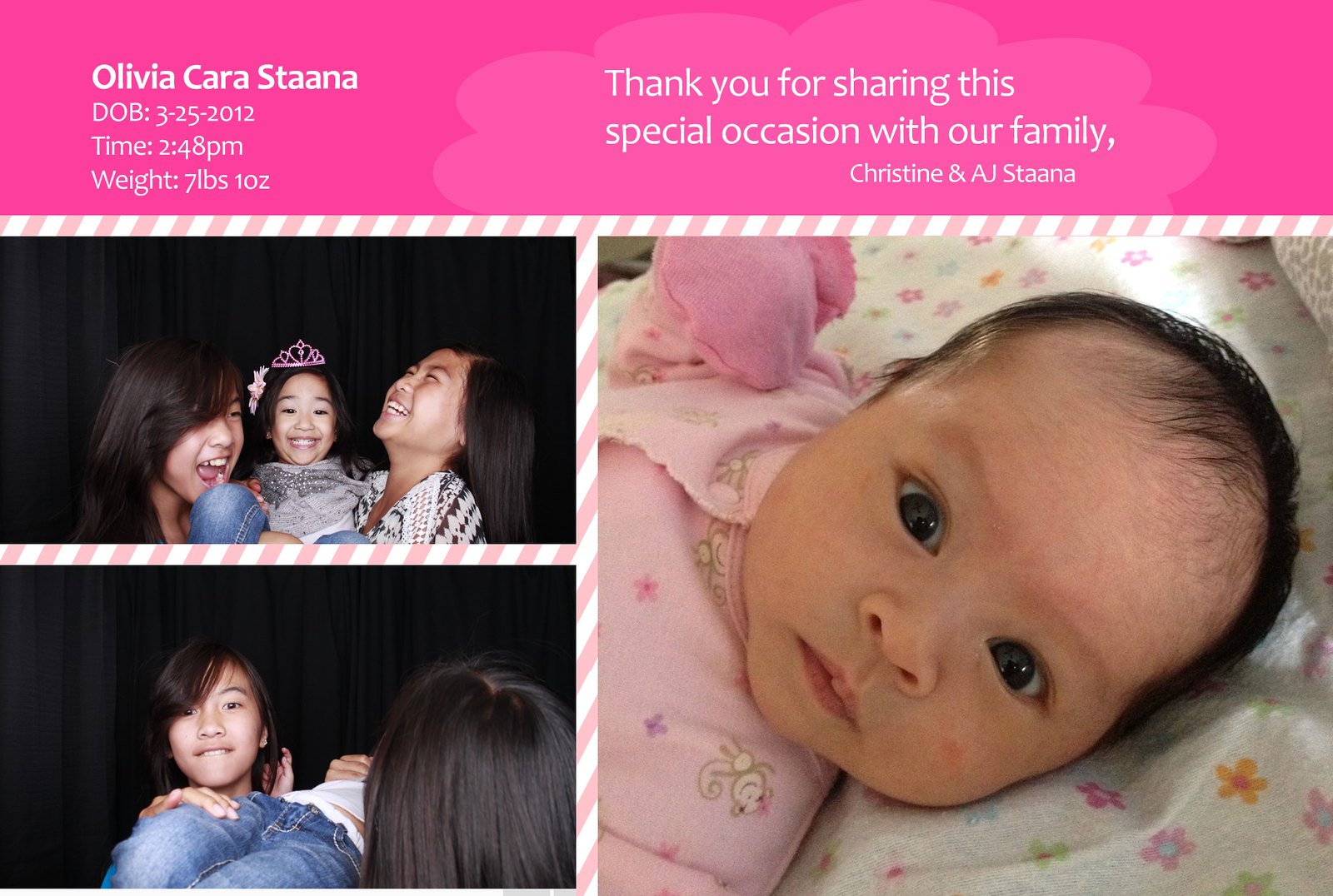The image resembles a postcard and is centered around a family announcement. At the top, there is a bright pink banner featuring white text that reads: "Olivia Cara Stana, Date of Birth: 3-25-2012, Time: 2:48 PM, Weight: 7 pounds 1 ounce." To the right of this text is the message: "Thank you for sharing this special occasion with our family, Christine and AJ Stana." 

Below the banner, the background showcases a combination of colors including various shades of pink, white, gray, tan, blue, and black. The bottom half of the image contains three photographs: on the left, there are two vertically stacked photos of what appears to be a group of young girls. The first photo shows them laughing against a black backdrop, while the second photo provides a closer crop, focusing on one of the girls. On the right, there is a larger color photograph of a baby with dark hair, wearing a pink printed onesie and pink mittens, lying in a crib adorned with a flowered blanket. The overall style and setting present a joyous family celebration, capturing intimate moments and festive elements.